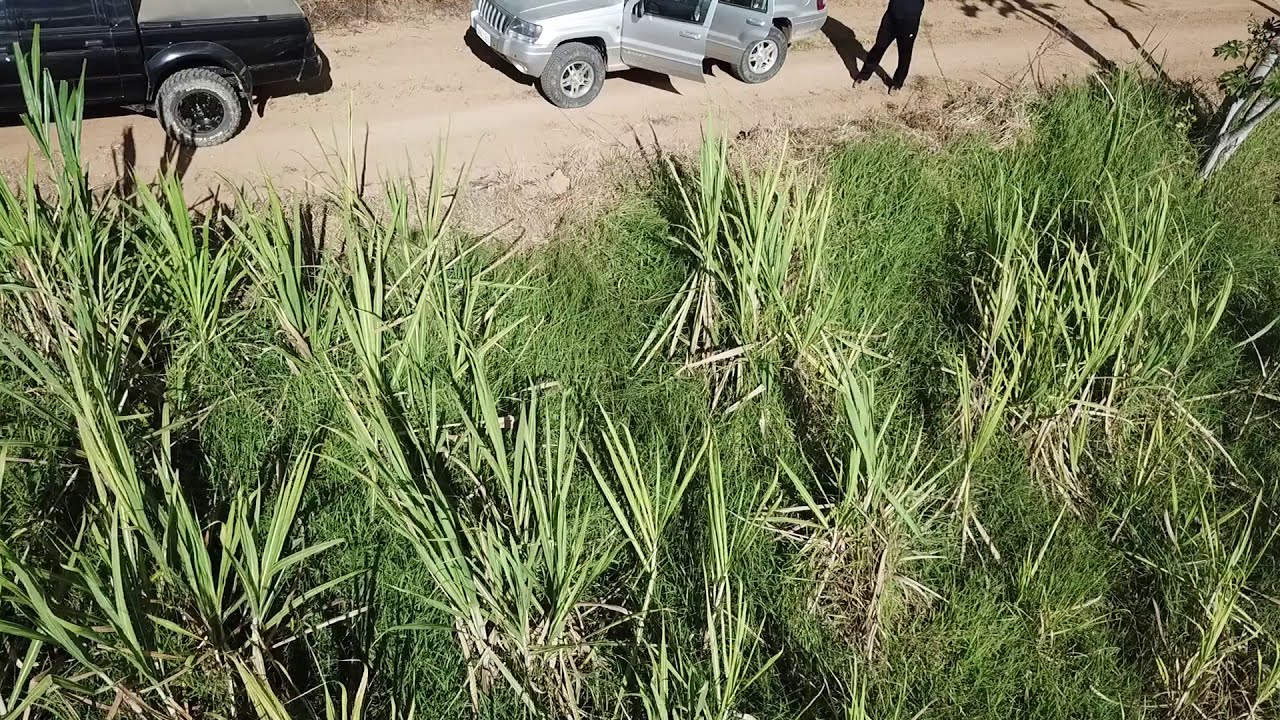The color photograph, captured in landscape orientation from a downward drone perspective, showcases a partial landscape scene. In the foreground, a grass-covered hill is dotted with spiky plants resembling the tops of palm trees, minus the ferns, their narrow leaves about three to four feet long. Above this grassy area, a horizontal dirt road cuts across the top of the image. On the road, partially visible in the left corner, is a black pickup truck with black rims. Central to the image is a silver Jeep Wagoneer with both its driver's side and passenger side doors wide open. Next to the Jeep, a man dressed entirely in black—pants, shirt, and shoes—is seen from the chest down, facing the camera. The photograph captures a realistic and detailed aerial view of this serene yet dynamic roadside scene.